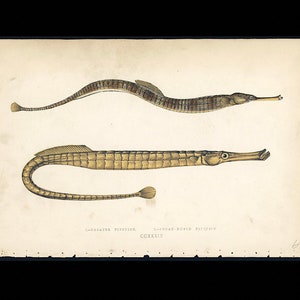The illustration depicts two elongated, eel-like creatures reminiscent of needlefish or sea snakes, possibly some ancient animals. Both creatures have a pronounced beak-like snout, constituting around 20% of their body length, and fish-like eyes with puffy cheeks behind them. The top creature sports alternating brown and white stripes along its body and has an S-shaped curve. In contrast, the bottom creature is a solid golden yellow, with its body curving into a J shape and ending in a feature reminiscent of a tassel or ball at the tip of its tail. They are set against a creamy background with some text at the bottom, which is too small to decipher.